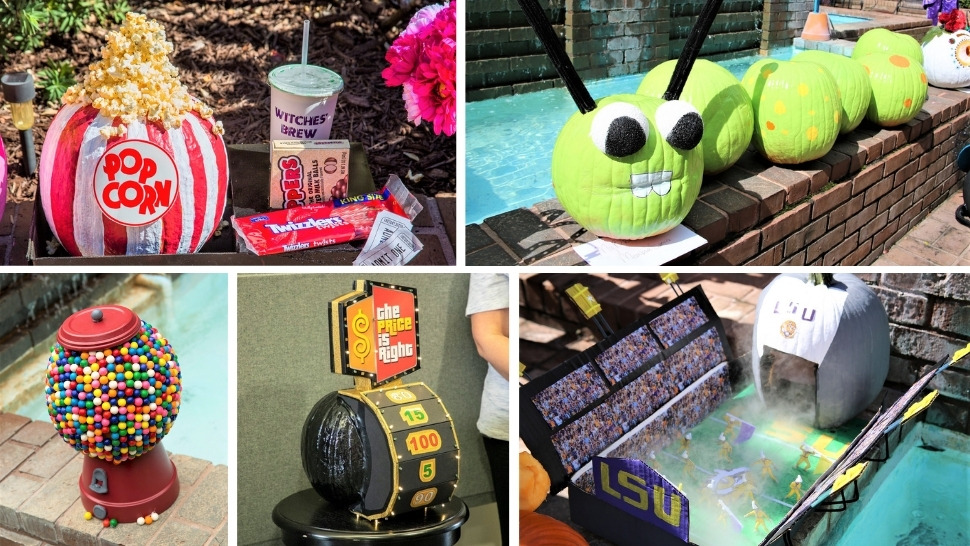This collection of illustrations consists of five distinct images, each bordered with a white outline. In the top left box, there is a movie-themed snack setup, featuring a spherical popcorn bucket, a soda cup labeled "Witch's Brew," a box of Whoppers, some Twizzlers, and two movie tickets. To the right of this, the next box displays a whimsical caterpillar made from five green-painted pumpkins, complete with glued-on eyes, a painted smile, and small horns, all perched on a brick wall beside a swimming pool. Below the snack setup, the bottom left box contains a gumball machine also positioned on a brick wall near a pool. In the center of the bottom row is a miniature version of the spinning wheel from "The Price is Right," displaying the show's logo at the top. The bottom right box showcases an overhead view of a detailed diorama depicting an LSU football stadium, complete with model players on the field and a photograph of spectators surrounding the representation of the seating area.